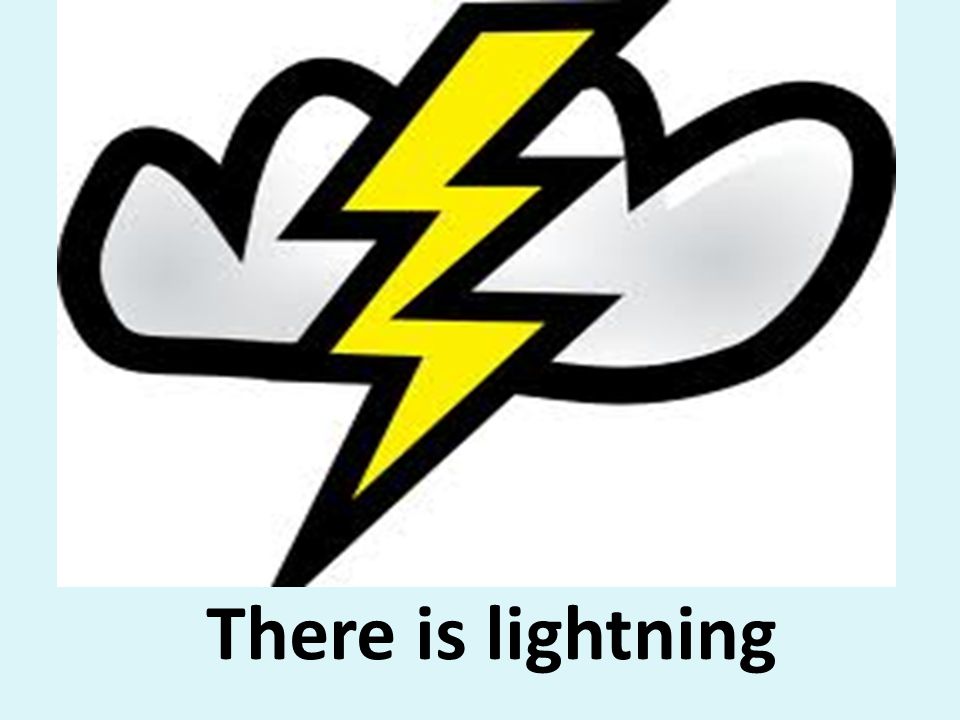This clipart image features a vivid yellow lightning bolt with three jagged edges, prominently positioned in the center. The lightning bolt is sharply outlined with bold black lines, giving it a well-defined and striking appearance. Behind the lightning bolt is a stylized white cloud, also outlined in black, with four rounded peaks at the top to convey a fluffy texture, and a flat bottom edge. The overall background of the image is white, but a light blue border frames the left, right, and lower sections, forming an almost U-shaped outline. At the bottom of the image, within this light blue border, centered in large black text, it reads "There is lightning." This crisp and clear illustration could easily serve as a visual alert in a weather application or website, warning viewers of potential lightning, indicating they should stay indoors to avoid the associated dangers.